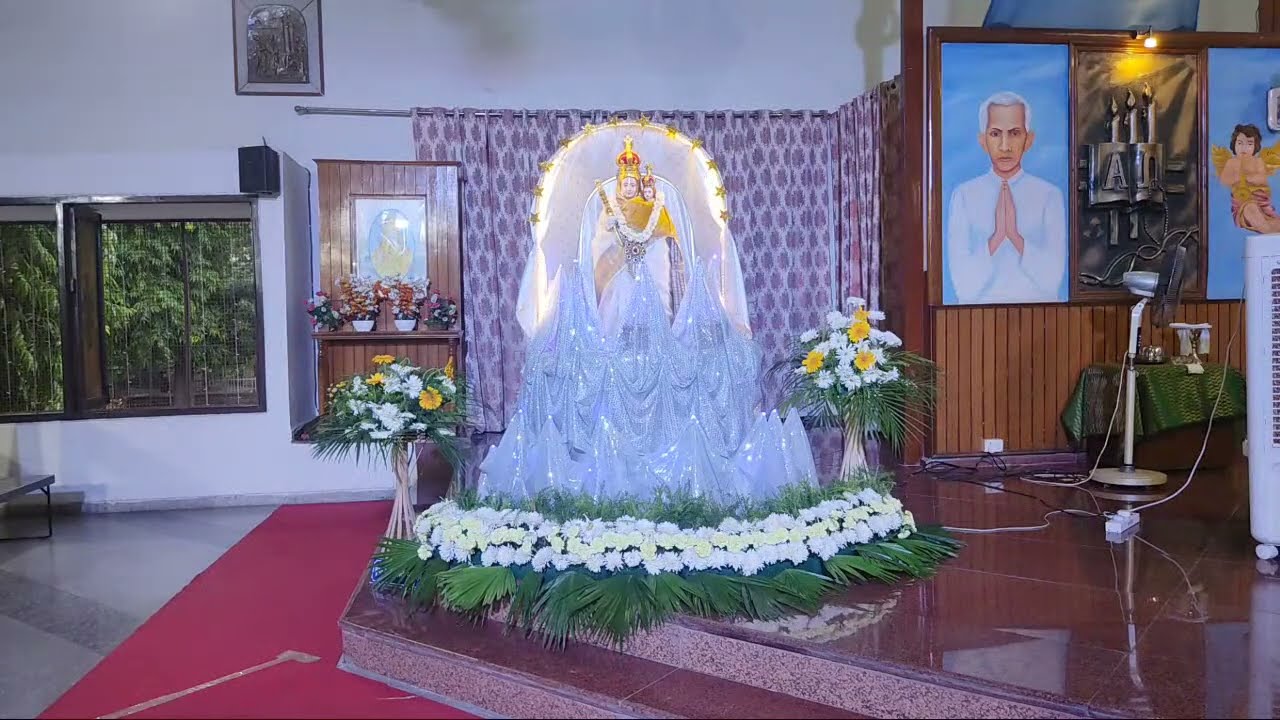This photograph depicts a detailed religious ceremony taking place on a stage. At the forefront, a seamless burgundy marble floor transitions into steps leading up to a stage adorned with intricate arrangements. At the base of the stage, a circle of palm leaves is meticulously laid out, topped with a row of pristine white flowers. Adjacent to these arrangements, bowls containing white and yellow flowers add vibrant touches.

The centerpiece of the stage features a Hindu deity in yellow attire with a striking red crown. This deity, adorned with a garland of white flowers and draped in flowing blue and white fabrics, stands commandingly on a pedestal. Flanking the deity is a smaller figure, both enveloped by rich, burgundy-patterned curtains.

To the viewer's right, a wooden paneled wall displays a poignant painting of a man with white hair and a white shirt, hands clasped in prayer against a blue background. Nearby, a three-dimensional artwork resembling a metal book with candles accentuates the religious ambiance.

Overall, the image communicates a sacred, reverent atmosphere, enriched by detailed decor and religious iconography, all painstakingly arranged to honor and elevate the solemnity of the ceremony.